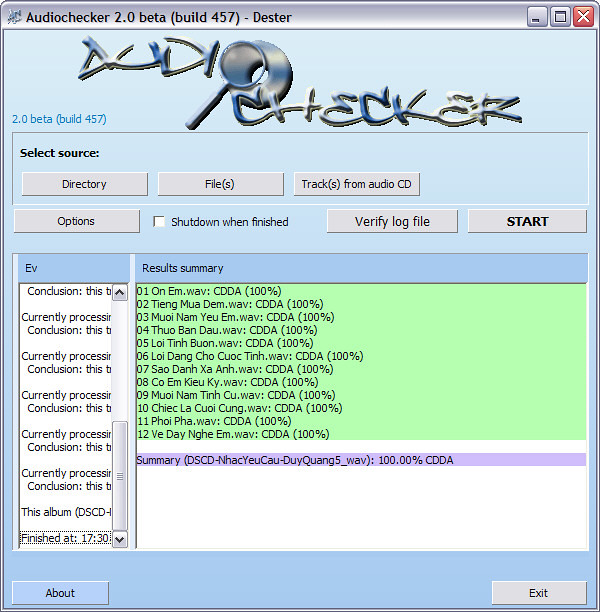The image displays a software window titled "Audio Checker 2.0 Beta (Build 457)" at the very top, with standard Windows icons for closing, minimizing, and maximizing the window to the top right. The page has a light blue background, with segments in white, green, and blue. Below the title bar is the "Audio Checker" logo, featuring a stylized magnifying glass where the circle forms the "O" in "Audio." 

The page content is organized with a white area displaying buttons labeled "Directory," "File," "Track from Audio CD," "Options," "Verify," "Log File," and "Start," all in small gray rectangles with black text. Underneath, there's a "Results Summary" section on a light green background, listing different .WAV files, predominantly showing 100%. 

Further down, a light purple section contains another summary with similar 100% indicators. To the left, there is a thin sidebar repeatedly saying "currently processing," running from the center-left to the bottom-left of the image. At the bottom-left, there's an "About" button and, at the bottom-right, an "Exit" button, set against the persistent blue background. Overall, the interface combines computer-themed font and visual elements specifically tailored for this audio verification software.